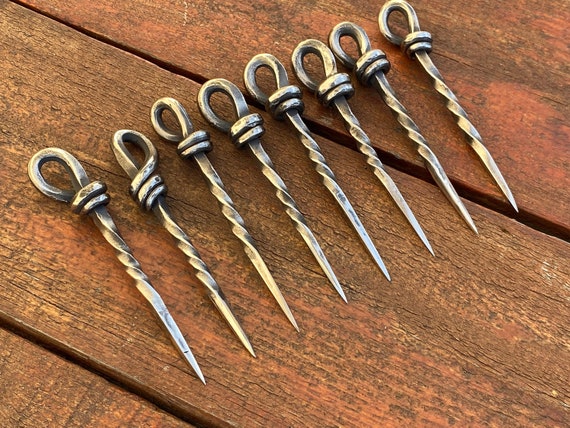The image shows eight intricately designed metal hooks with a rustic patina, neatly lined up side-by-side on a wooden surface. Each hook features a rounded top that loops into two or three decorative swirls, followed by a long, spiraled shaft that tapers into a pointed end. The metal appears unpolished, displaying darker marks that add to their rugged charm. The wooden surface they rest on has a reddish-orange stain, resembling a deck or table, and provides a warm contrast to the metallic tones. The pointed ends of the hooks are aligned and directed toward the bottom right of the image. Although the exact purpose of these hooks is unclear, their consistent design and careful arrangement suggest they could be tools meant for digging or anchoring, possibly used in outdoor activities like setting up tents.